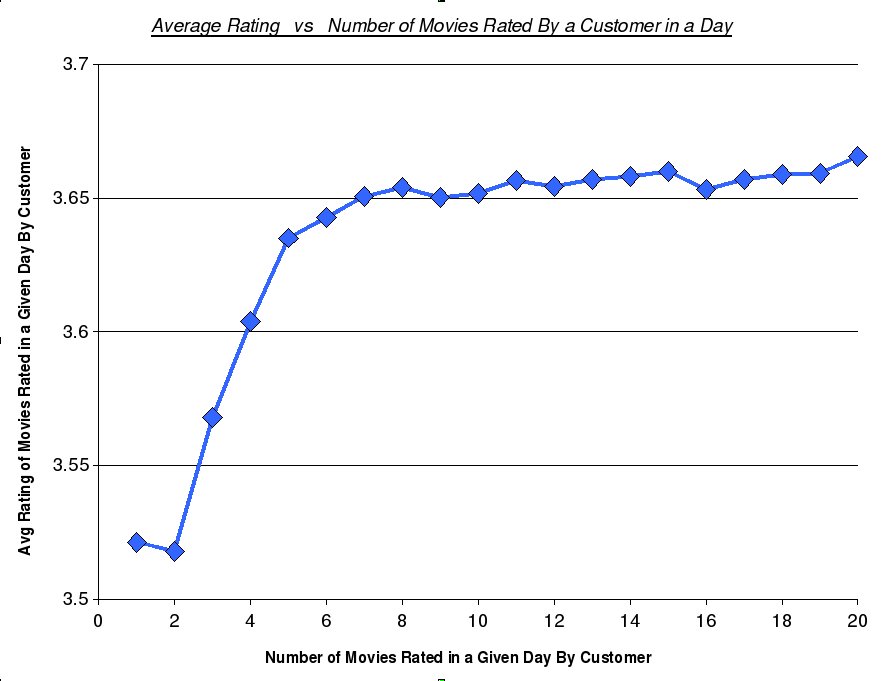The image is a line graph set against a white background, featuring blue plots and data points. The title of the graph reads "Average Rating Versus Number of Movies Rated by a Customer in a Day." The x-axis is labeled "Number of Movies Rated in a Given Day by Customer" and ranges from 0 to 20 movies. The y-axis, labeled "Average Ratings of Movies Rated in a Given Day by Customer," ranges from 3.5 to 3.7. 

Initially, the average rating starts slightly above 3.5, but around the point where the number of movies rated reaches 2, there is a sharp increase. Beyond this initial surge, the graph shows that the average rating levels off, fluctuating slightly but predominantly staying between 3.65 and 3.7 from the 4 to 20 movie mark. The presentation is straightforward, lacking source attribution or additional context, making it somewhat challenging to interpret fully.